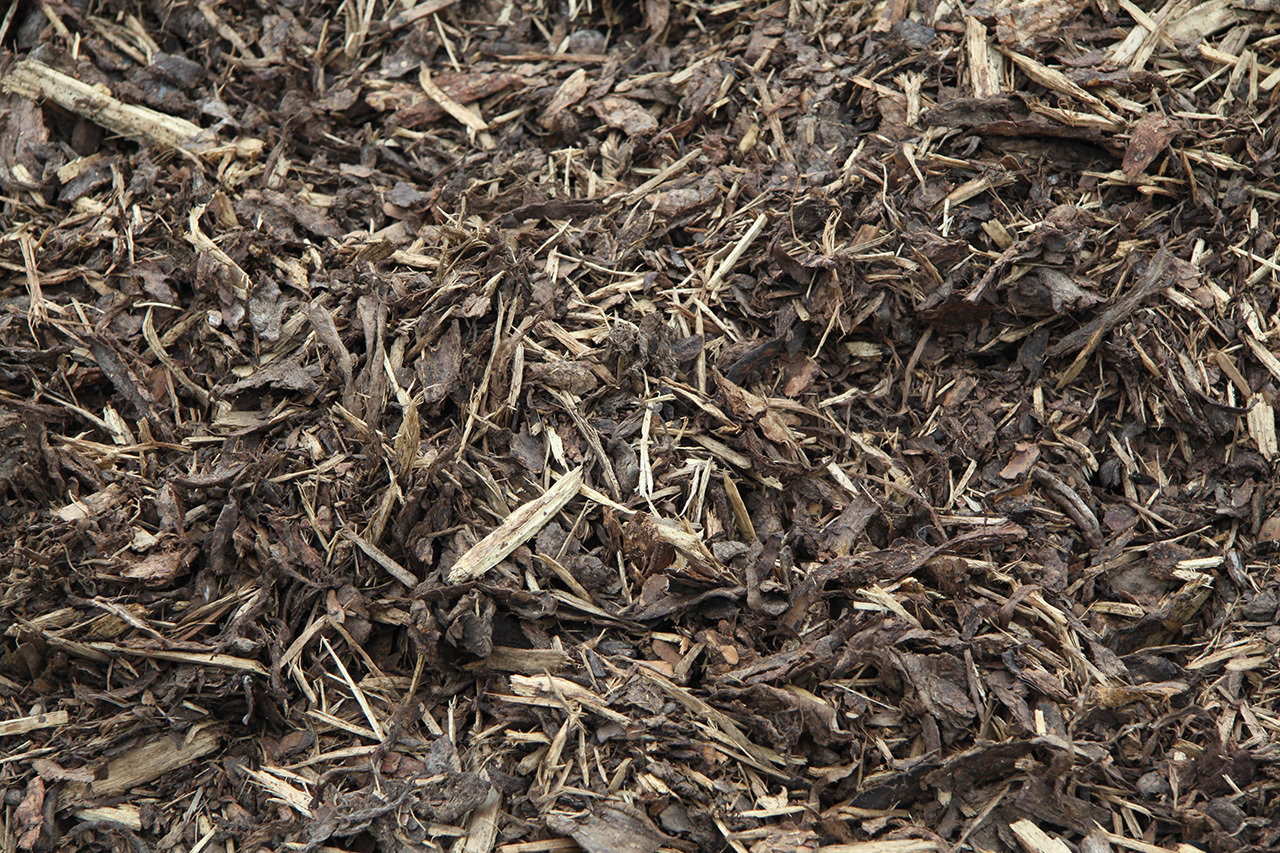The image is a landscape-oriented color photograph depicting a closely-packed view of mulch, consisting mainly of small wood chips and twigs, in various shades of tan and dark brown. Captured from a height of about a foot above the ground, the photo fills the entire frame with fragments of wood and dead grass, scattered evenly across the scene. The tightly-packed clippings, featuring both larger stick-like pieces and finely chopped mulch, extend from edge to edge, with a couple of light beige blades of grass near the center and a noticeable twig in the top left corner. The setting appears to be outdoors, with a naturalistic, representational approach that emphasizes the varied textures and colors found in the organic material lying flat on the forest floor.